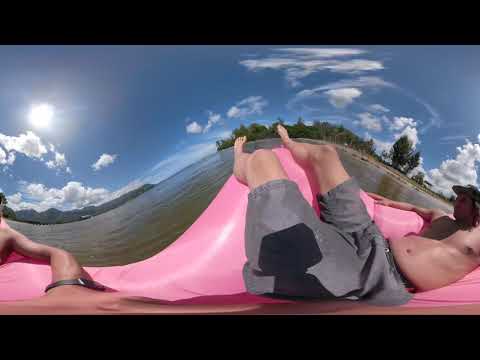The image, taken with a highly distorted, fish-eye-like lens, captures an outdoor scene under a sunny, blue sky dotted with fluffy white clouds. The main subject in the foreground is a shirtless, white-skinned male wearing a hat and gray swim trunks, reclining on a pink inflatable floaty on what appears to be a lake. The water lacks the clarity typical of the ocean, suggesting it is indeed a lake. To the left, only parts of another person, possibly a male, are visible—an arm and a leg—adding an element of mystery. The distorted, wavy appearance of the image causes the surroundings to appear uneven and surreal. In the background, the landscape features trees and distant mountains, adding to the serene yet peculiar atmosphere.